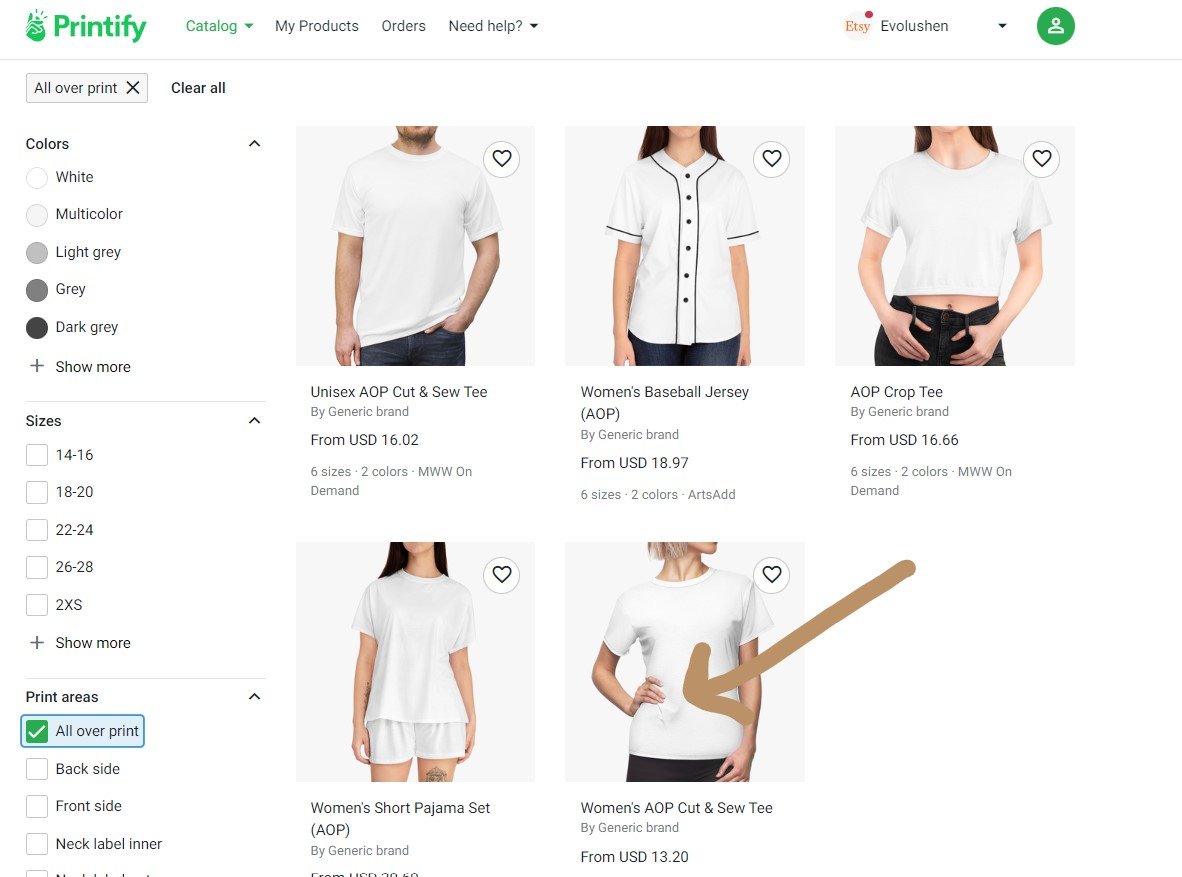The image displays a detailed interface from the Printify platform, showcasing a variety of customizable apparel options. The interface features two main tabs highlighted in green: "Printify" and "Catalog". Other options include "My Products", "Orders", and "Need Help". 

There are various visual elements, such as a gray circle with the Etsy logo in red, and another icon representing "Evolution" as a green circle with a white profile icon. 

Below the header, there are product listings for different types of apparel:

1. A man wearing a white shirt labeled as "Unisex ALP Cut and Sew Tee", priced from USD 16.02. It is available in six sizes and two colors. Provider: MWW On Demand.
2. A woman in a white shirt with black buttons, referred to as "Women's Baseball Jersey (ALP)", priced from USD 18.97. It also comes in six sizes and two colors. Provider: Arts Ad.
3. A girl wearing a white cropped shirt, labeled as "ALP Crop Tee", with a starting price of USD 16.66. Available in six sizes and two colors. Provider: MWW On Demand.
4. A woman in a white shirt with a brown arrow pointing to it, listed as "Women's ALP Cut and Sew Tee", starting at USD 13.20.

Each product detail includes options for size and color variations depicted by circles matching the respective shades: white, multi-color, light gray, gray, and dark gray. The listing interface also includes an expandable section indicated by a plus (+) symbol to show more details.